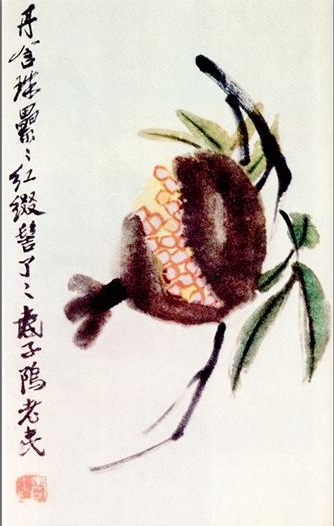This image displays a detailed Asian-style painting on a long white panel. Dominating the left side, there is a column of black Chinese calligraphy that extends vertically, concluding with a prominent red Chinese stamp at the bottom. The foreground features a central brown, rounded object, suggestive of a cut-open fruit or nut, revealing a cluster of small white pearls or seed pods with an orange outline. Surrounding this central element are subtle hints of yellow coloring. A short black branch with four or five elongated green leaves extends into the composition, adding to the botanical theme. The background remains stark white, emphasizing the simplicity and elegance of the painting's design.